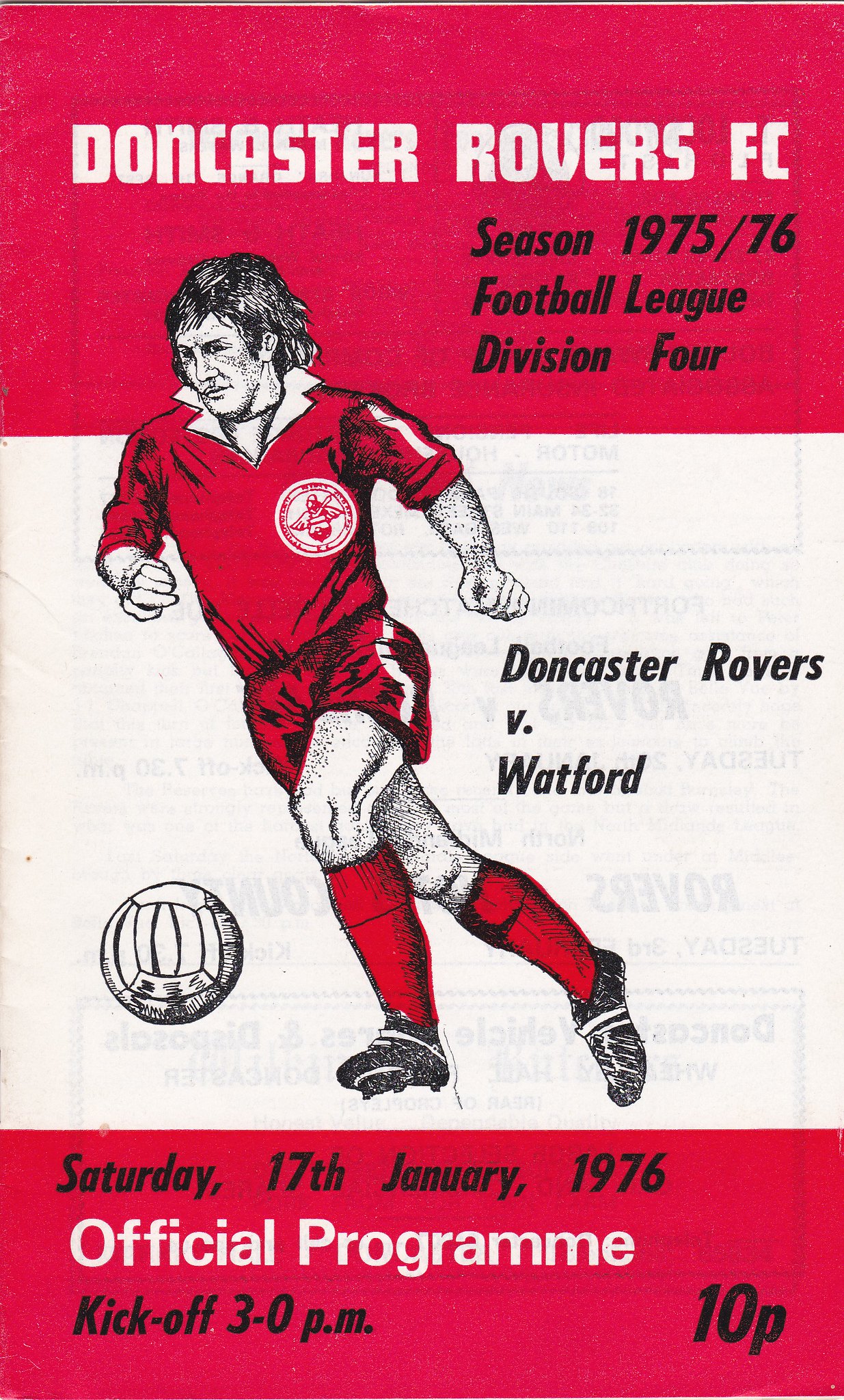This image is a scan of an advertising flyer or program cover for a Doncaster Rovers FC soccer match. The top section features a striking red background with "Doncaster Rovers FC" in bold white letters. Below this, aligned to the right, the text details the "Season 1975-76, Football League, Division IV" in black. Centrally placed is a white banner showcasing an illustration of a soccer player in a red jersey and socks, positioned in a forward running stance with a ball at knee level, poised to kick. To the right of the illustration, in black text, it reads "Doncaster Rovers v Watford." At the bottom, another red banner displays "Saturday, 17th January 1976" in black, followed by "Official Program" in prominent white letters. Below this, in smaller black print, it notes "Kickoff 3:00 PM." The price "10p," presumably indicating 10 pence, is placed in the bottom right corner in black.